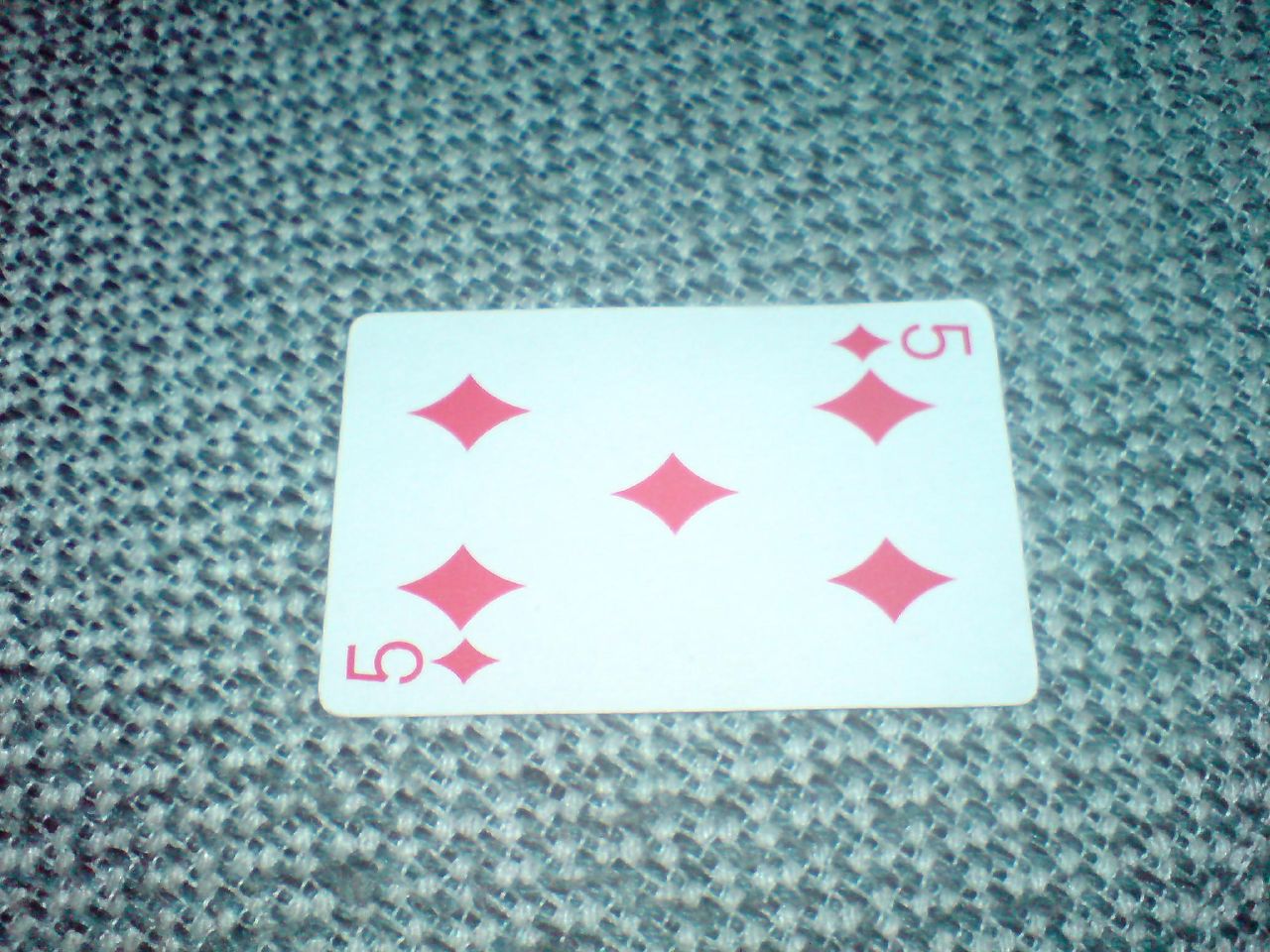This close-up photograph focuses on a single playing card from a deck, centrally positioned within the frame. The card is laid horizontally on a light blue and black patterned carpet, which serves as the background, creating a subtle yet contrasting backdrop. The card is a white five of diamonds, displayed face up. Due to the horizontal orientation, the numerals and smaller diamond symbols in the bottom left and top right corners appear sideways. In addition to these corner embellishments, the card features five larger red diamond symbols: two at the top, two at the bottom, and one precisely in the center. There are no additional markings or numbers on the card, making it the sole focus of the image. The detailed close-up emphasizes the simplicity and symmetry of the five of diamonds.